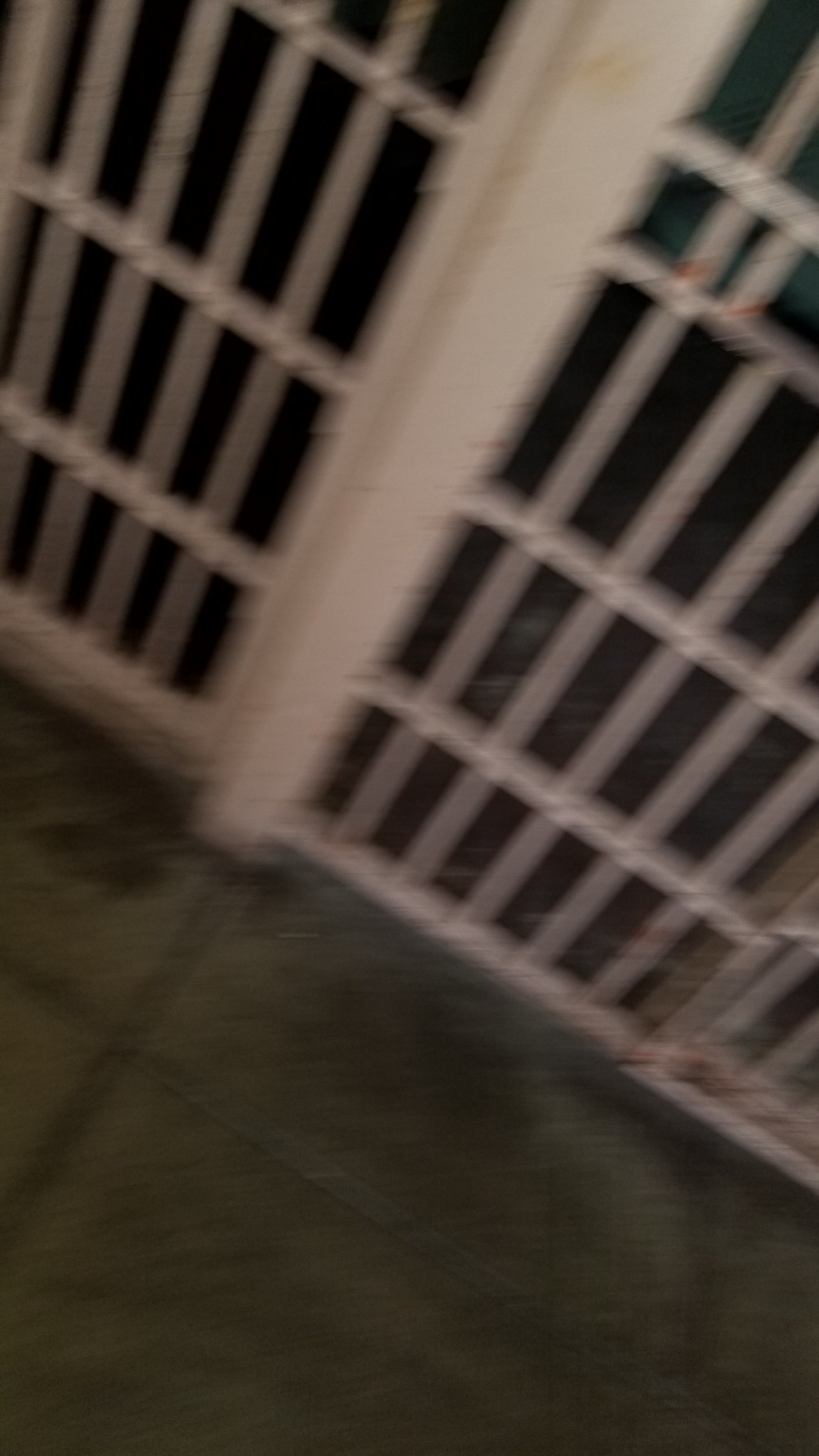This image, taken from outside looking through a blurry metal cage or jail cell, primarily focuses on the lower portion of a cage door. The cage itself is constructed from criss-crossing metal bars painted white or beige and is reinforced with a thick vertical metal bar, as well as an L-bracket joining the segments. The scene is dimly lit, suggesting it might have been captured at night. The ground is a dark, unclean concrete floor made up of large, stone slabs with masonry in between. Scattered debris hints at neglect. Beyond the cage bars, the background fades into darkness, adding to the overall eerie and dismal atmosphere of the scene.